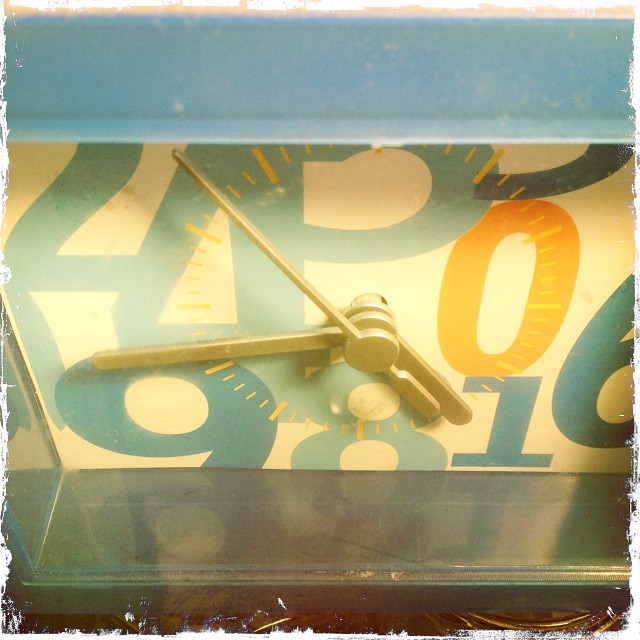The image features a clock with an unconventional design. The numbers are color-coded and scattered around the clock face: the number 2 is light blue, the numbers 9 and 1 are dark blue, the number 8 shares the light blue shade of the number 2, and the number 0 is a striking orange. These numbers are not part of the actual clock face but seem to be separately placed. The clock face itself consists of a series of short and long lines, with the longer lines indicating where the numbers traditionally would be. The clock has three hands: a short hour hand, a longer minute hand, and a thin second hand. At this particular time, the hour hand points to the 5, the minute hand to 41, and the second hand is at 52 seconds, indicating the time is 5:41:52. The clock is bordered by a blue rim at the very top, adding a touch of color to its overall appearance.